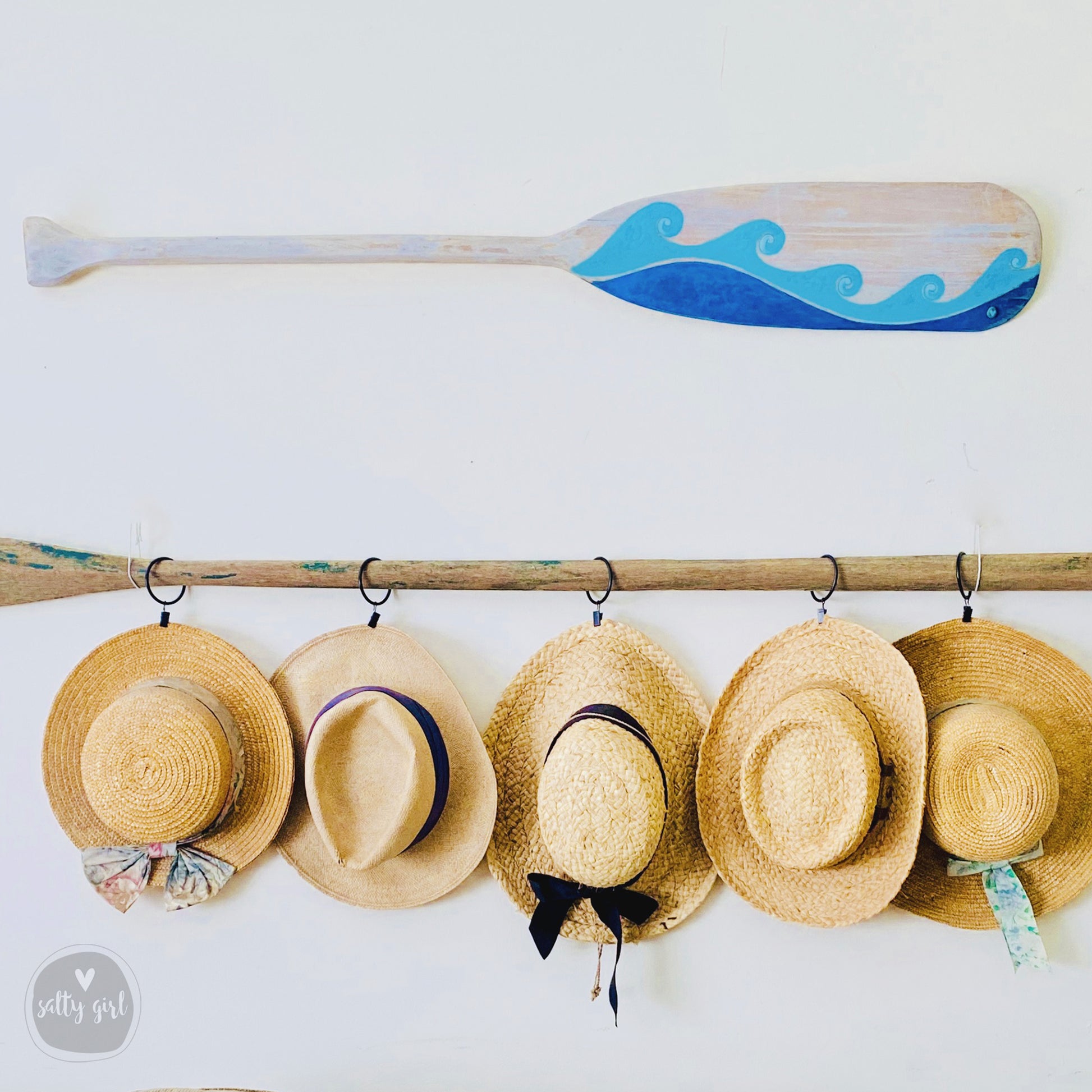The image features two boat oars mounted on a stark white wall. The top oar is a shorter white one, painted with a blue wave design, featuring a curved dark blue section below lighter rolling blue waves. The entire oar is visible, with the paddle on the right and the handle on the left. Below the painted oar hangs a longer, mostly brown oar with remnants of blue or green paint, partially stripped. This oar holds five straw hats, each hung by black circular hooks. The hats are embellished with decorative bands and bows; three have bows while two are banded without bows, suggesting different styles. In the bottom left corner, the logo "Salty Girl" with a heart emblem is displayed.